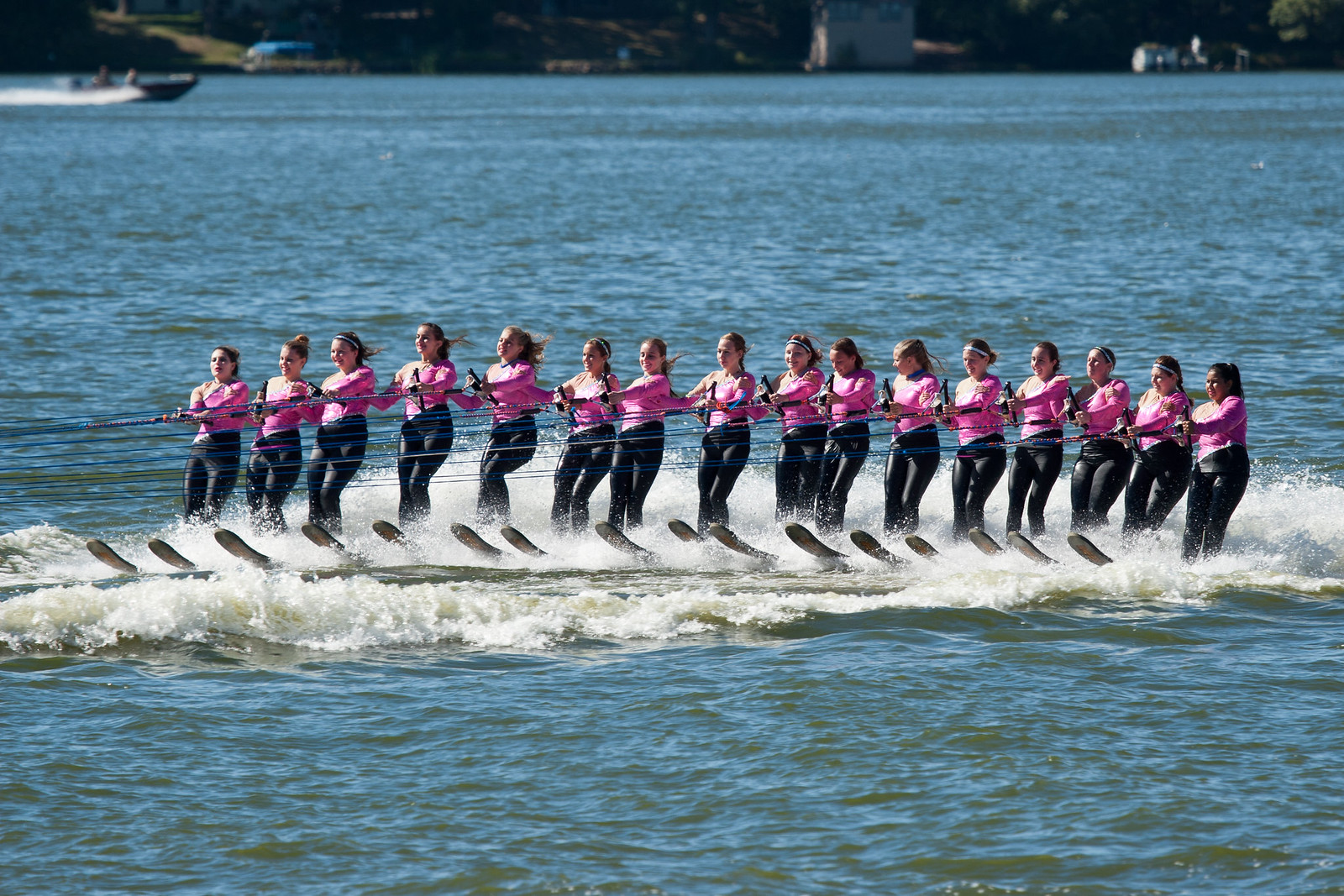In this photograph, a group of approximately 15 women are water skiing in close formation on a calm lake. Each skier wears a matching outfit consisting of long-sleeved, hot pink tops and black pants. Their hair is neatly tied back in ponytails or buns. The women hold onto ski ropes being pulled by a boat in front of them, creating noticeable wakes and splashes in the water. The serene backdrop of the image showcases a tranquil lake with trees lining the distant shore. The scene captures the dynamic energy and coordination of the skiers as they engage in this synchronized water sport.